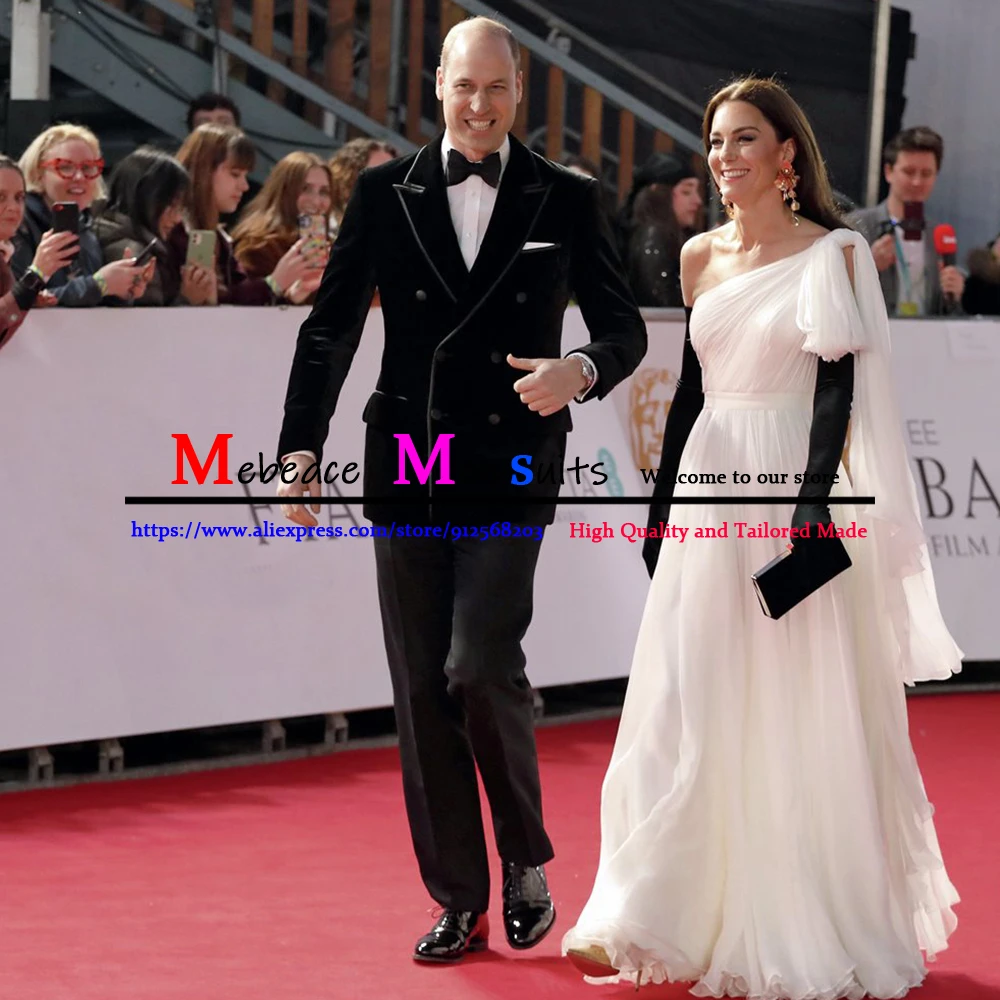This photograph captures Prince William and Princess Kate elegantly walking down a red carpet. Princess Kate is dressed in a sophisticated white gown paired with long black gloves, holding a black clutch purse, and accessorized with long dangling earrings. Her brown hair cascades down her shoulders, complementing her pale skin and warm smile. Prince William is by her side, donning a black velvety tuxedo featuring a velvety jacket, a black bow tie, a crisp white dress shirt, and shining black shoes. He is partially bald and also smiling. A crowd of onlookers stands behind a banner, taking photos with their smartphones, while a staircase can be seen in the background. Additionally, a partly visible script overlays the image, referencing "Misfits: Welcome to Our Style" with a URL link to a high-quality, tailor-made clothing store.